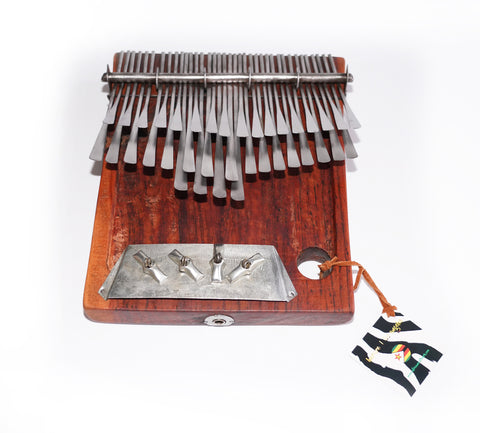The image depicts a thick, square wooden board with a reddish-brown, rough surface adorned with black streaks and cut marks. Positioned on a bright white background, the board features a circular hole in the lower right-hand corner where a brown leather tag is attached. The tag bears a black and white zebra print label, and additional intricate details, such as a yellow-red flag with a star, are noted. Across the top of the board runs a shiny steel bar supporting dozens of skinny, flat metal tabs, resembling typewriter keys but without imprints. Below this arrangement, there's a shiny gray metal plate with metallic elements sticking out, which appear to be part of a mechanical device or possibly a series of long, triangular-shaped spoons or keys. The scene is intricately detailed, suggesting an elaborate and somewhat enigmatic apparatus atop the wooden board.